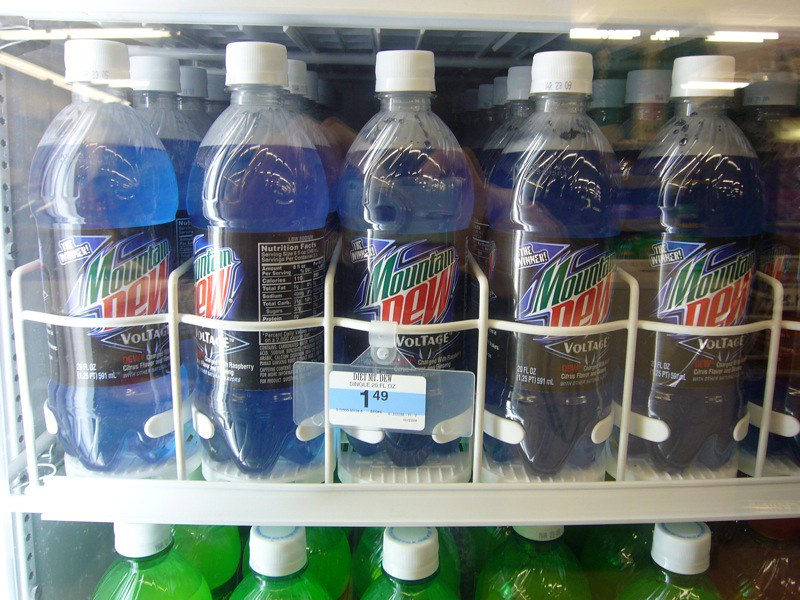The photo depicts a fully stocked retail store cooler, showcasing neatly arranged rows of Mountain Dew Voltage and what appears to be traditional Mountain Dew. The primary focus is on the five visible rows of Mountain Dew Voltage, with each medium blue soda in clear, 20-ounce plastic bottles featuring white twist-off lids. The cooler holds multiple rows extending back behind each front bottle, indicating a robust inventory. The price tag in the center of the display reads $1.49. Just below these blue sodas, the tops of green-capped, clear bottles suggest the presence of traditional green Mountain Dew in a similar five-row configuration, though less visible. The entire setup resembles the typical soda aisle found in convenience stores like 7-Eleven, with pristine, eye-level shelving.